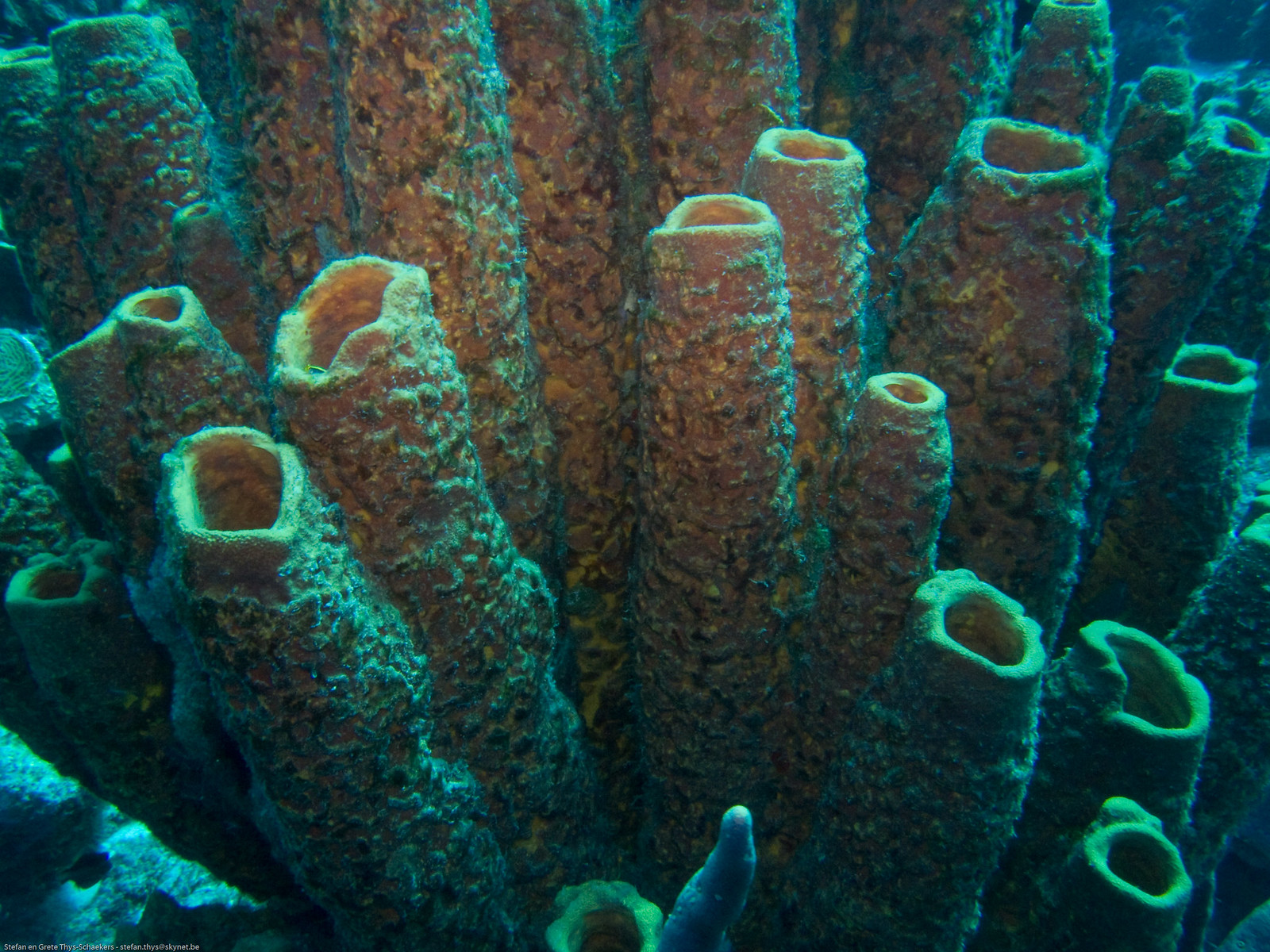The photograph, taken in landscape format and rich in subtle underwater hues, vividly captures the intricate textures of towering underwater chimneys, commonly found near geothermal vents on the ocean floor. These chimneys, rising to an estimated height of two feet, are formed over time through the stacking of volcanic carbon and sulfur substances, though they appear to have ceased their activity as no emissions are visible. The scene is bathed in a bluish-green glow, characteristic of deep-sea environments, which softens the palette, blending the original tan and off-white colors of the chimneys. Among these cylindrical structures, each with an opening at the top, a small, distinctive piece of blue coral stands prominently at the bottom center of the composition, contributing to the overall serene and mysterious marine landscape.